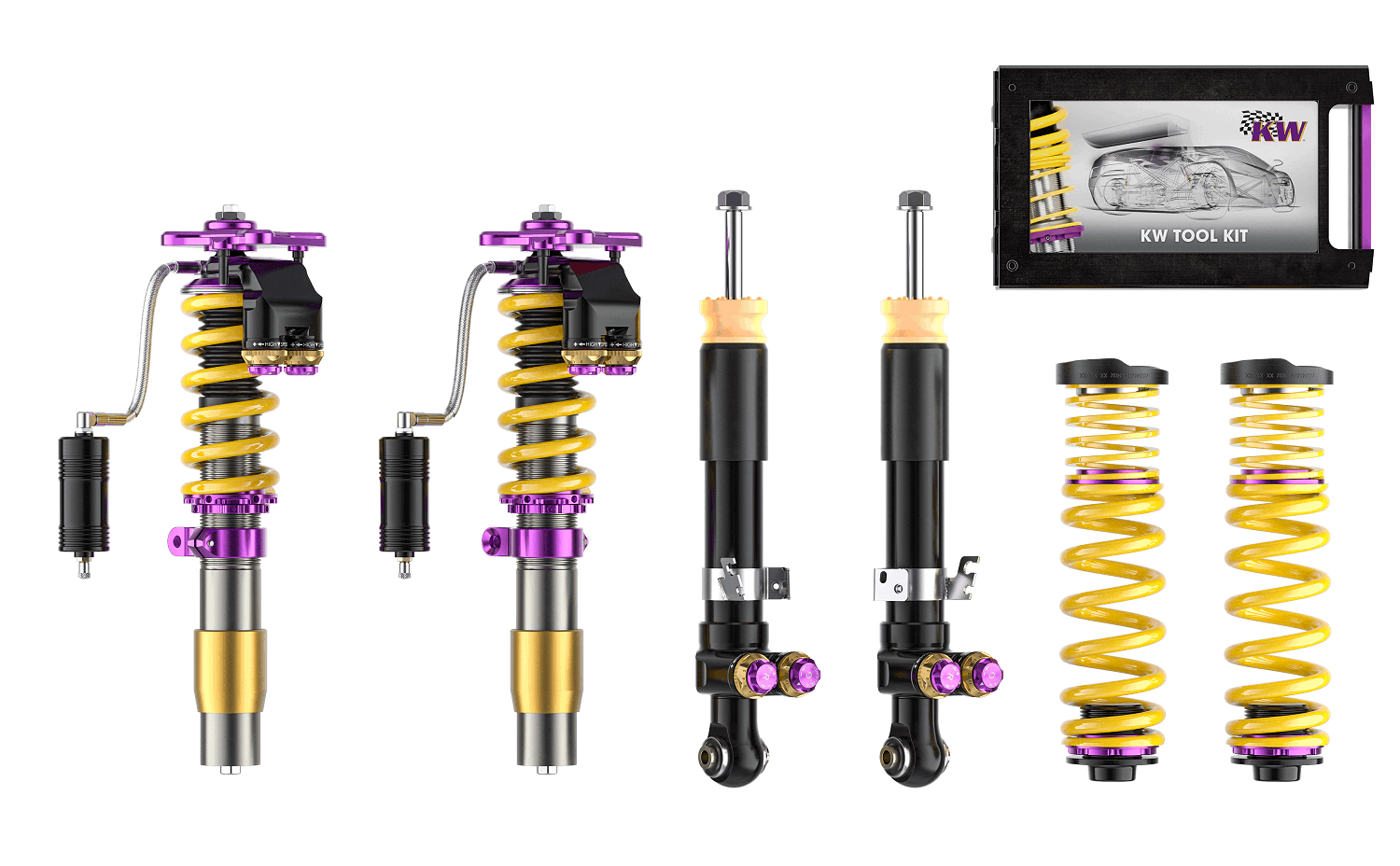The image depicts an advertisement for the KW Toolkit, prominently showcasing a variety of specialized tools. Central to the display are pairs of twin tools that appear to be shock absorbers, characterized by their circular metal cylinders and cranks on the side. The springs, visible in bright yellow, are highlighted with connectors in contrasting purple and gold metal. On the left side of the image, two apparatuses with spiral yellow wires extend from silver and gold bases to the top, featuring an input portion for installation. The upper right corner contains a black-bordered box with a gray background labeled "KW Tool Kit," prominently displaying the KW symbol and brand name. Additionally, two yellow spiral tubes with screws at the bottom and caps at the top are positioned under the box, while the center features two black, rounded, tubular tools with silvery tops resembling screws, contributing to the toolkit's comprehensive presentation for automotive or mechanical fine-tuning.